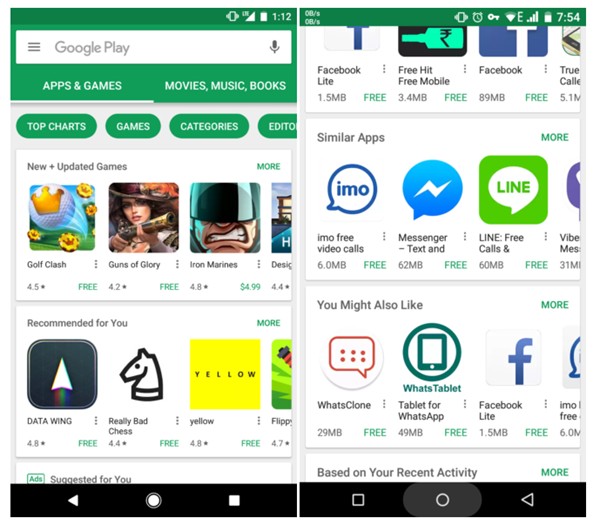The image showcases two screenshots from a mobile device displaying different sections of the Google Play Store:

1. **First Screenshot**:
    - **Header Section**: A prominent green bar displaying "112" on the left.
    - **Search Bar**: A white search bar featuring a microphone icon, indicating voice search capability.
    - **Navigation Tabs**: Tabs labeled "Apps & Games" (underlined), "Movies & TV," "Music," and "Books."
    - **Category Navigation**: Light blue boxes labeled "Top Charts," "Games," "Categories," and "Editor's Choice" in green.
    - **Featured Games**:
        - "New & Updated Games" section highlighting:
            - "Golf Clash"
            - "Guns of Glory"
            - "Iron Marines"
            - An unnamed game partially visible.
    - **Additional Games**: White boxes listing "Data Wing" and "Really Bad Chess" in yellow, along with another partially visible game.
    - **Advertisements**: An "Ads" section labeled "Suggested for You."
    - **Navigation Bar**: A black bar at the bottom with triangle (back), circle (home), and square (recent apps) icons.

2. **Second Screenshot**:
    - **Header Section**: Green bar displaying "754" on the left.
    - **Featured Apps**:
        - "Facebook Lite"
        - "Free Mobile"
        - "Facebook"
        - Another partially visible app.
    - **Similar Apps**:
        - A white box listing:
            - "IMO Free Video Calls and Text"
            - "Messenger"
            - "LINE Free Calls & Messages"
          (with another app cut off)
    - **Recommendations**:
        - "You Might Also Like" featuring:
            - "What's Clone"
            - "Whats Tablet"
            - "Facebook Lite"
            - Another app not fully visible.
        - Recommendations are based on recent activity.
    - **Navigation Bar**: A black bar at the bottom with square, circle, and triangle icons.